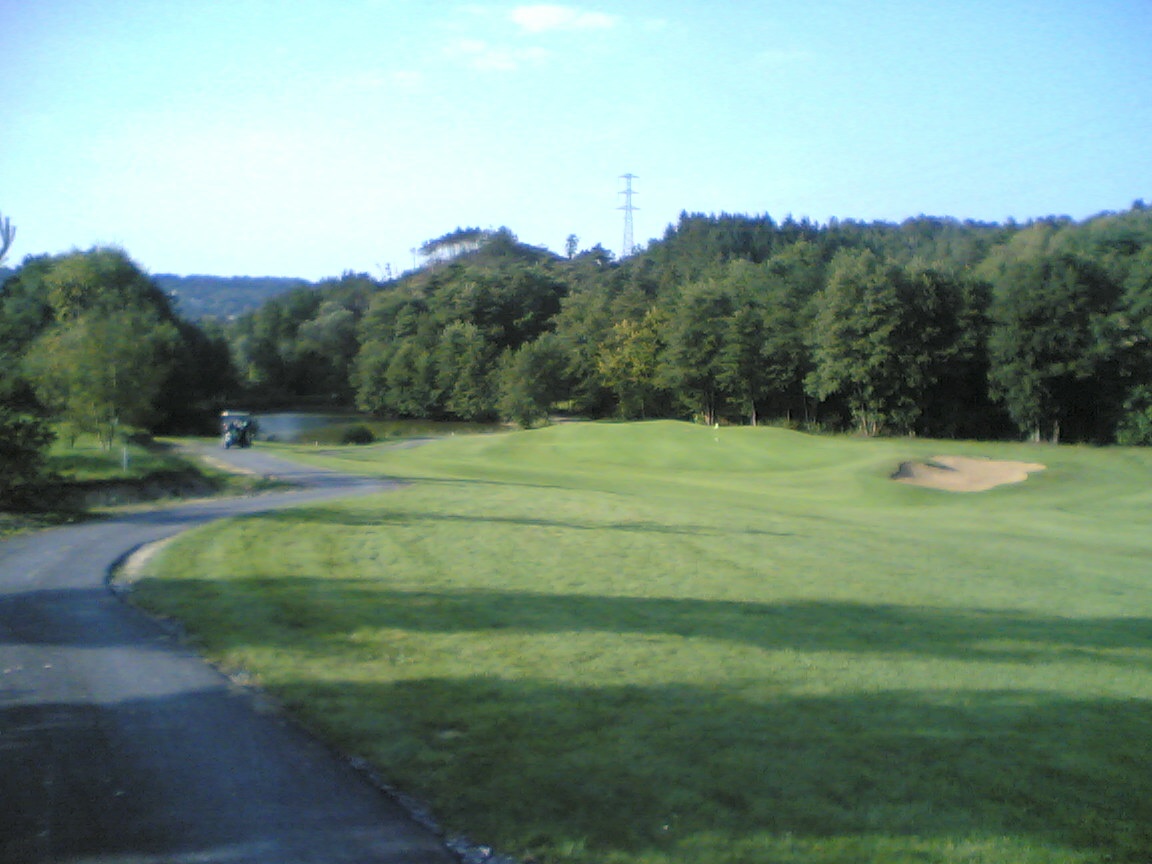This slightly blurry, color photograph captures an outdoor scene in the middle of a sunny day on a golf course. At the center of the image, a paved golf cart path winds through the landscape, leading to a white golf cart positioned slightly to the left. To the right of the path, the vibrant, green fairway features a small yellow flag and a sand pit. The terrain is mostly flat with a hint of undulating hills, all covered in lush, manicured grass devoid of weeds. Thick, bushy trees frame the background under a sky that is lightly sprinkled with white clouds. An electric power pole stands tall and prominent towards the distant background, adding an industrial touch to the serene setting. The photograph doesn't include any text or identifying markers, making it a quintessential, timeless capture of a leisurely golf course scene.